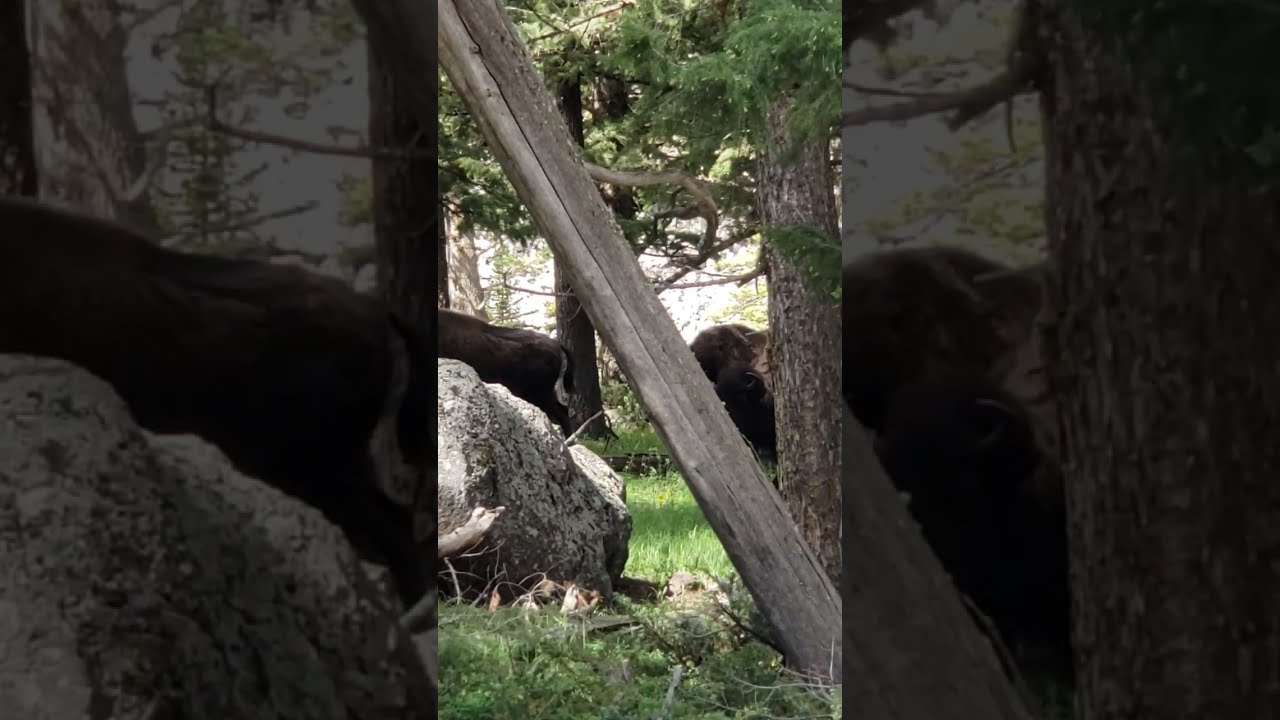This daytime outdoor photo appears to be taken in a wooded area, possibly within a zoo exhibit. Central to the image are two black animals that resemble bears, although they could also be mistaken for cows or hippos due to their size. One animal is near a large boulder, partially obscured, while the other is positioned towards the far right. A diagonal fallen log, likely an old cedar tree trunk, stretches from the top left to the bottom right corner, adding a sense of natural texture to the scene. A prominent pine tree with lush green needles and multiple branches stands in the background, along with additional tall trees, contributing to the forested setting. The ground is covered in green grass with some scattered twigs and dead limbs in the foreground. The overall color palette includes various shades of green, gray, brown, and white. The lighting suggests the photo was taken during the middle of a sunny day, allowing natural light to illuminate the scene. The entire composition brings a serene and detailed focus on the natural environment and the animals within it.